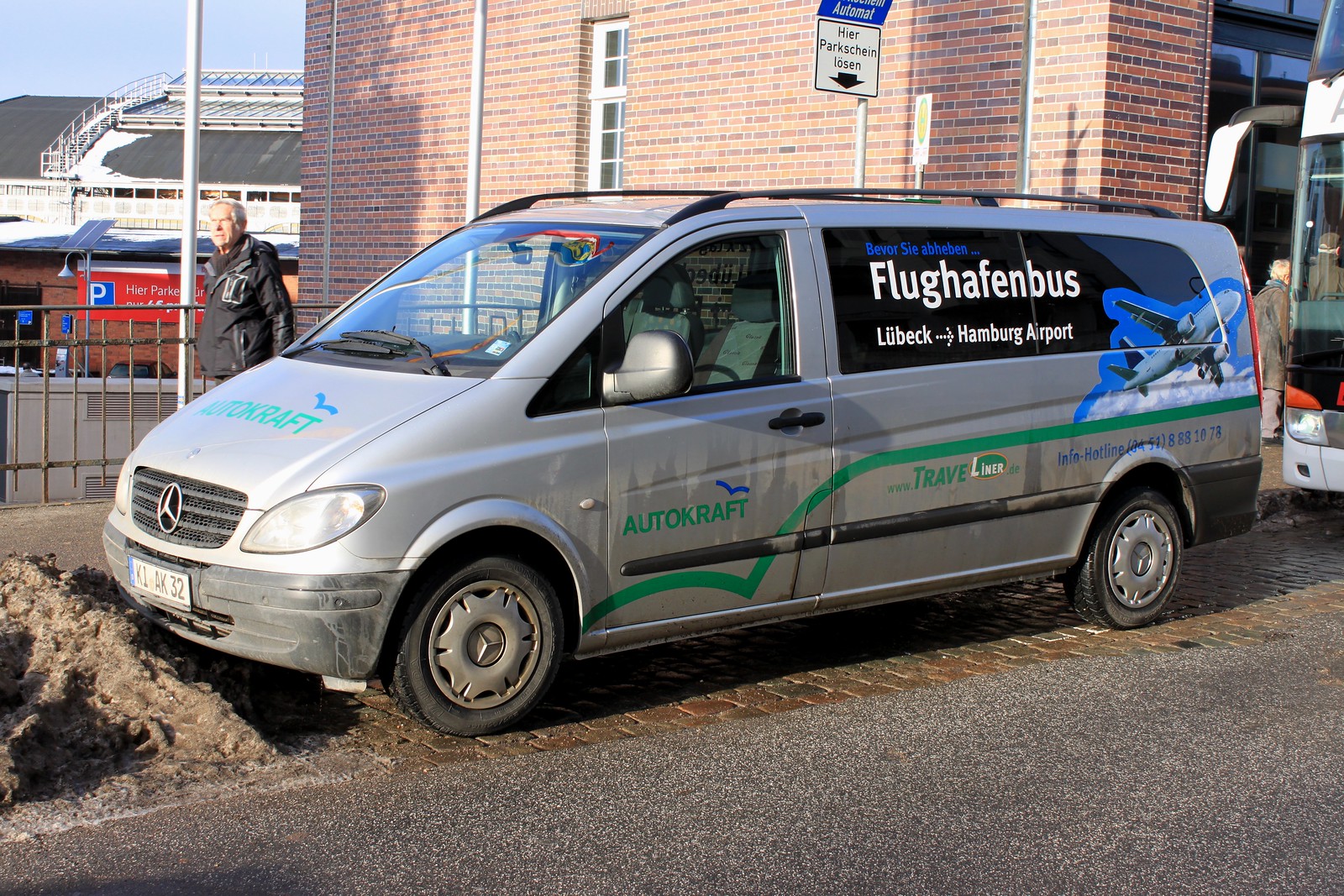In this detailed photograph taken in Germany, we see a gray van prominently parked in front of a brick building. The van, labeled with the brand "AutoCraft," features additional German text that reads "Flughafen Bus Lübeck Aero Hamburg Airport." This suggests the van functions as a shuttle service between the airport and various destinations. The side of the van displays a vivid graphic of an airplane against a heavy blue background, indicating its airport-related role. A man stands behind the van, and to the rear, a bus is visible with a man and a woman, presumably an elderly couple, seen through its window. Over the van, there are two signs: a white one immediately above it and a blue one farther up. The photo is taken from the street, focusing on the van as its central subject, with the partial view of what seems to be a blue and white ferry in the background, adding context to the scene's transportation theme.